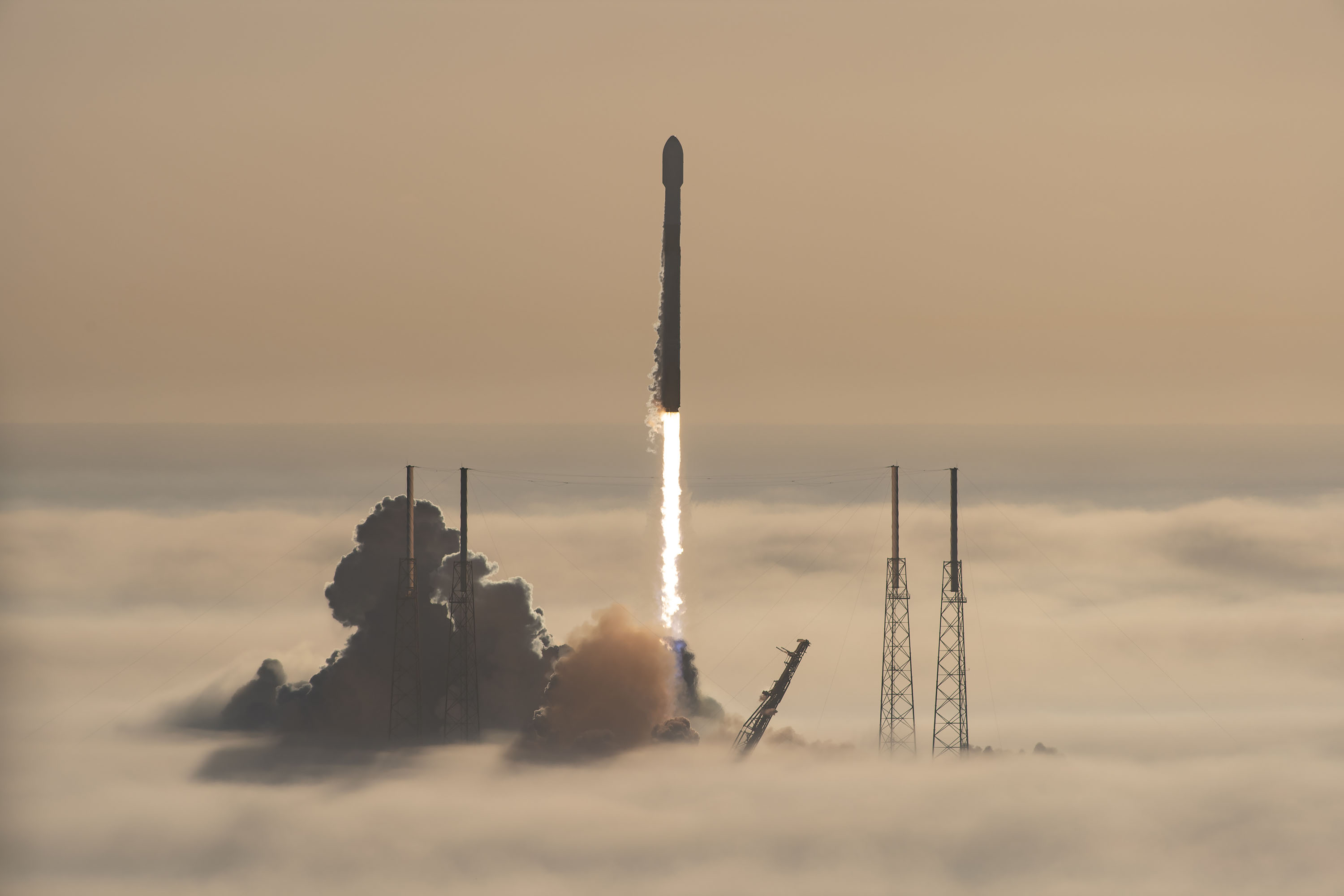In this hazy photograph capturing a rocket launch, the scene is set against a sky with shades of grayish pink, dark lavender, and hues suggesting either dawn or dusk. The focal point is a long, narrow rocket, distinguished by its shaft and head, lifting off with an intense streak of bright white light and jet fuel trailing from beneath. This powerful ascent is accentuated by a large orange cloud at the rocket’s base and additional billowing dark gray clouds flanking it on both sides. The launch site itself features metal towers, with one seemingly falling away as the rocket departs. The image encapsulates the dramatic intensity of the moment, with the ethereal lavender and pink hues of the clouds mingling seamlessly with the fog, creating a visually striking contrast of colors in the early morning or late evening sky.